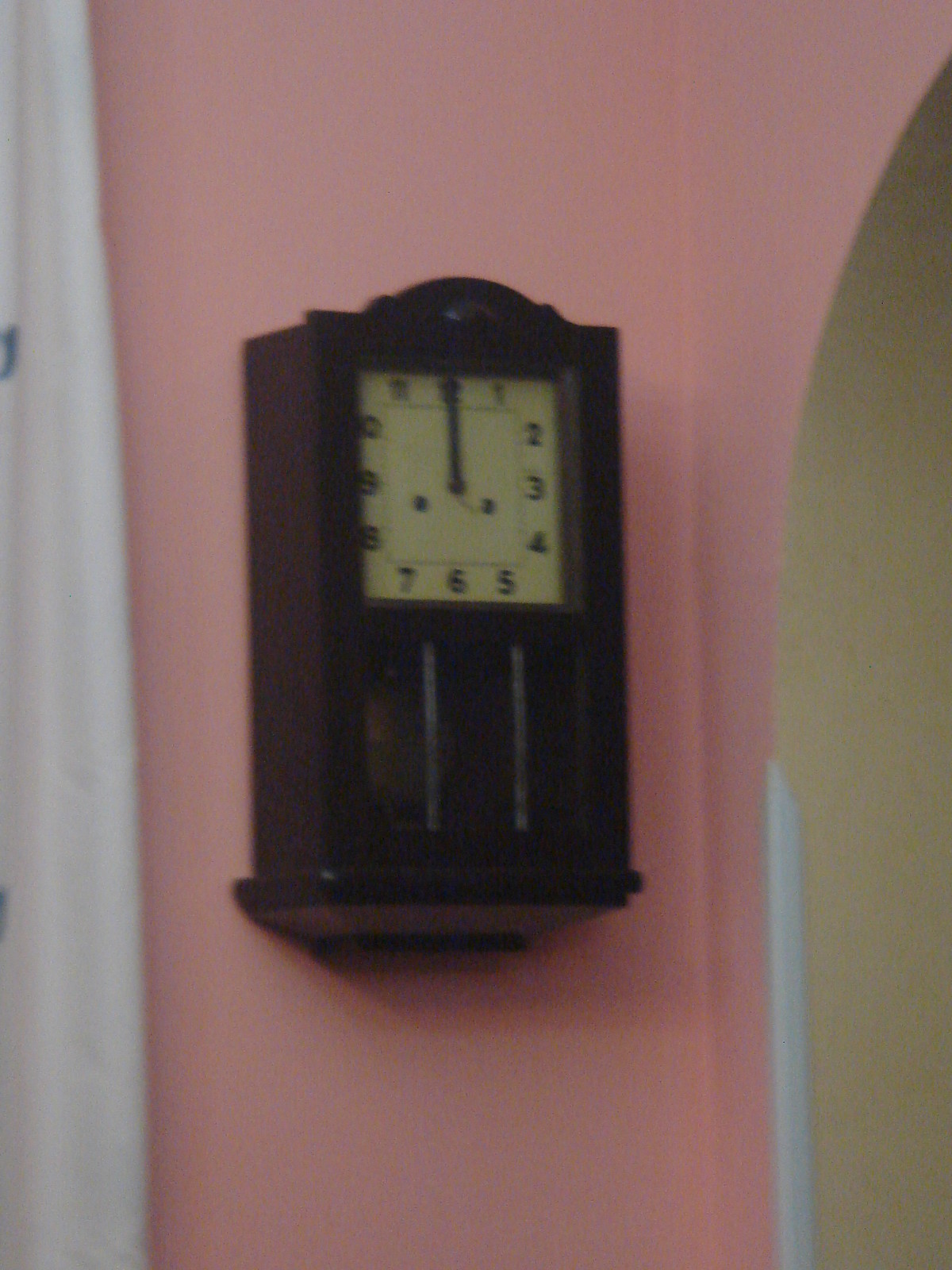This slightly blurry and grainy image, likely taken inside a house, captures a distinctive indoor scene. The photograph prominently features a pink wall alongside part of a pink archway. Mounted on the pink wall is a large, boxy clock, which appears to be either black or dark brown in color. The clock's rectangular form contrasts with its more usual round counterparts. The square clock face, occupying about half of the clock's front surface, is a pale yellow color and displays the numbers in a traditional circular arrangement despite the face's square shape. The hands of the clock are precisely set to 12 o'clock, right on the dot.